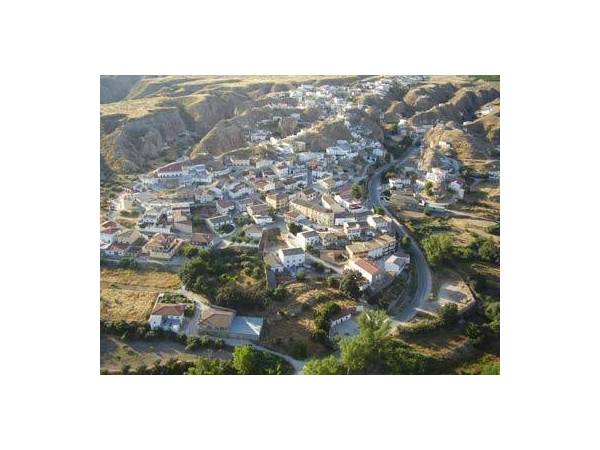This is an aerial photograph, possibly taken from an airplane, helicopter, or drone, capturing a small town nestled at the bottom of a mountainous valley. The town is composed of numerous white and gray buildings, some of which have dark gray roofs while others have reddish-brown or clay-shingled roofs. The buildings are arranged amidst yellow grassy patches and a central cluster of trees. A long winding road begins at the bottom center of the image, snaking its way along the right side, and eventually disappearing into the mountains. Smaller alleys and paths connect the various structures, although no people or vehicles can be seen due to the high vantage point of the photograph. Surrounding the town are agricultural fields, while imposing rock formations rise on both the top left and right sides of the image, casting subtle shadows across the landscape, indicating it is daytime.